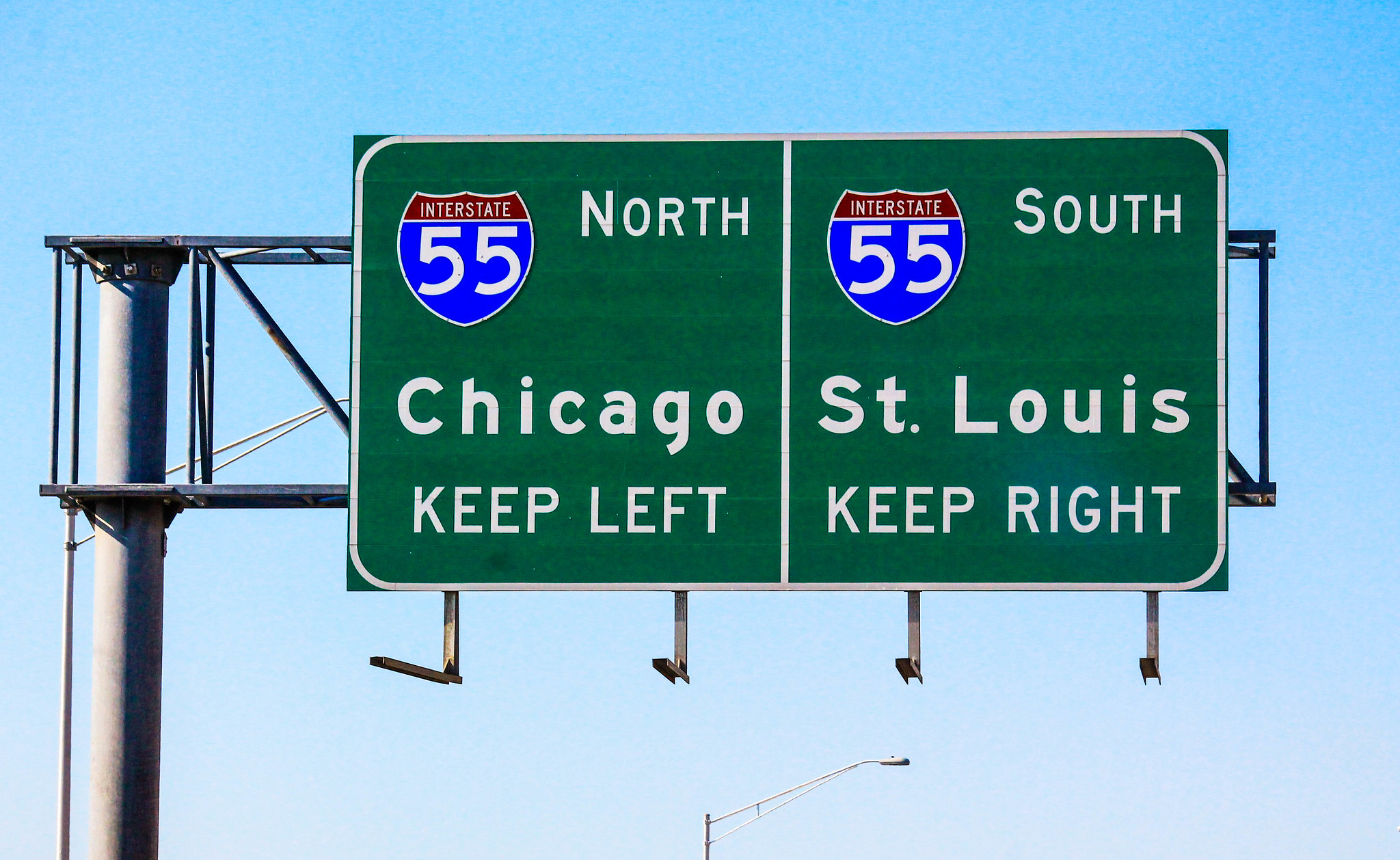This image captures a large green rectangular highway sign suspended over an unseen interstate, set against a daytime sky that transitions from dark blue at the top to lighter blue towards the bottom. The sign, attached to a substantial metal structure with a support beam on the left, features two distinct sections divided by a white vertical line. On the left side, it displays an insignia for Interstate 55 North, with "Chicago" underneath, instructing drivers to "keep left." The right side mirrors this layout but directs southbound travelers with an Interstate 55 South insignia, stating "St. Louis" and "keep right." Beneath the sign, a distant streetlamp pole is visible, along with four evenly spaced brackets that secure the sign to its structure.